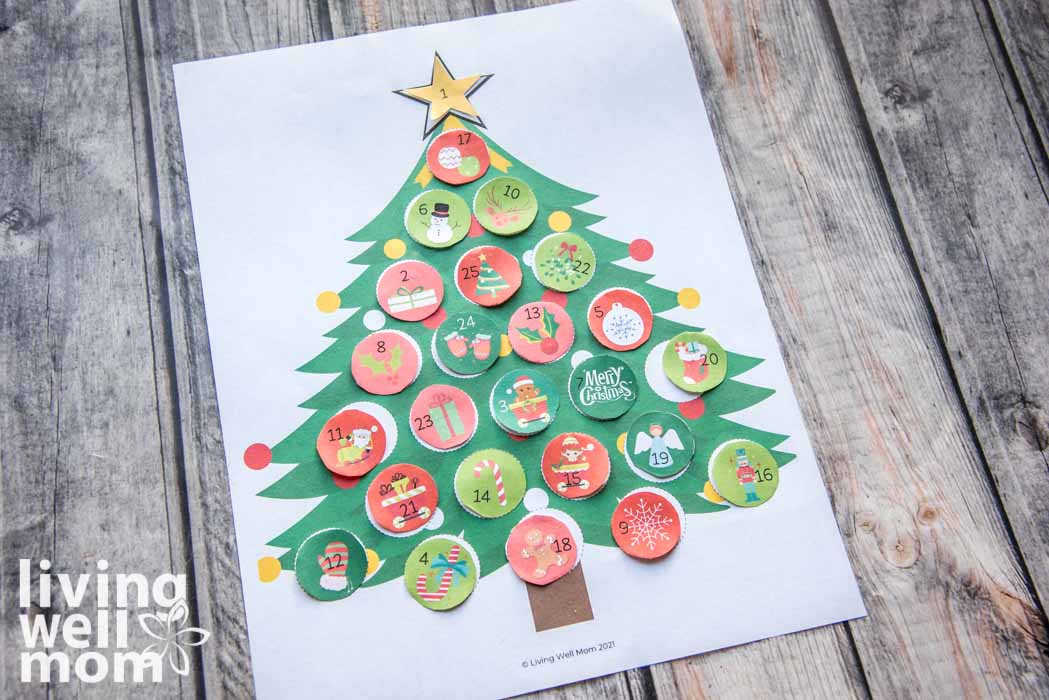The image is a professional color photograph depicting a Christmas advent calendar on a piece of paper, laying against long, realistic, grayish-brown hardwood floor planks. The calendar features a green Christmas tree with a brown trunk, adorned with various round ornaments. The ornaments and the yellow star atop the tree are numbered one through twenty-five, starting with number one on the star. Each ornament showcases different Christmas imagery and symbols including mittens, candy canes, wreaths, ornaments, snowmen, stockings, angels, snowflakes, gingerbread men, mistletoe, presents, reindeer, holly leaves, and some with text such as "Merry Christmas." The colors used are traditional holiday hues: red, green, black, white, gold, yellow, and brown. In the lower left-hand corner of the image, in bold white text, it says "Living Well Mom" with a small flower drawing. At the bottom of the tree, there is a copyright notice that reads, "Copyright Living Well Mom, 2021."